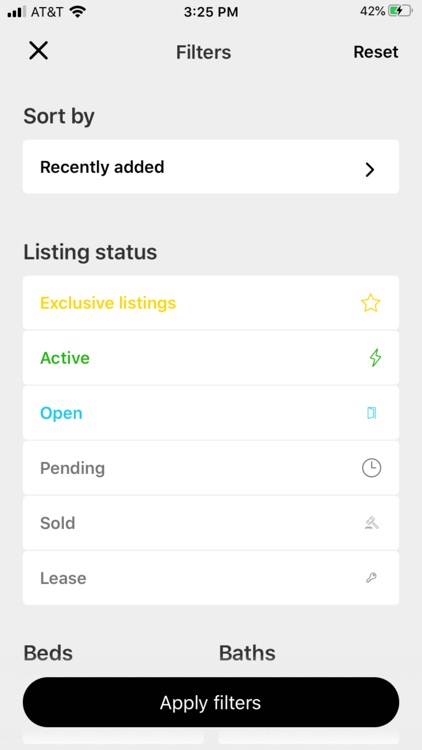This image is a detailed screenshot from either a phone or tablet interface, exemplified by the various status indicators and UI elements. 

In the top left corner, the network signal shows three out of four bars beside the "AT&T" label, alongside a full Wi-Fi signal. Centrally at the top, the time is displayed as "3:25 p.m." On the top right, a battery indicator reads "42%" with a charging symbol, a lightning bolt, and a green fill indicating its current level.

Below these status indicators, the interface reveals a navigation menu. Starting from the left, there is a close button represented by a cross (X), followed by a "Filters" option, and a "Reset" button. Directly beneath this row, a "Sort By" section appears with a white tab indicating the current sorting method as "Recently Added." An arrow on the far right of this tab suggests a dropdown menu for additional sorting options.

Further down, the "Listing Status" section is broken down into various categories, each distinguishable by color and iconography: 

- "Exclusive Listings" in yellow with a star icon
- "Active" in green accompanied by a green lightning bolt
- "Open" in blue with a door icon
- "Pending" in gray marked by a clock showing three o'clock
- "Sold" with a gray gavel
- "Lease" paired with a gray key

At the bottom of the list, there is another section labeled "Bids and Boths." Finally, the interface ends with a prominent black tab at the bottom, featuring the text "Apply Filters" in white, hinting at the functionality to apply the current filter settings.